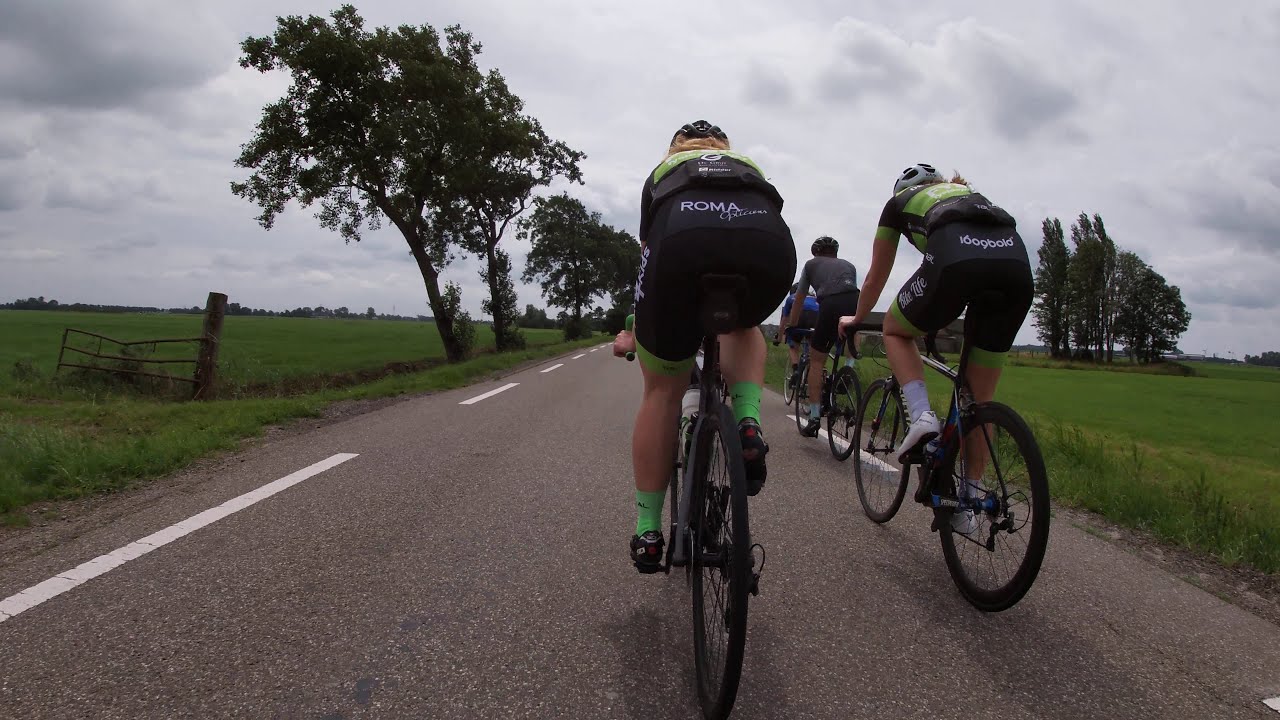This horizontally aligned rectangular photograph, taken during the day, features a group of bicyclists riding along a narrow, single-lane paved road. We are positioned behind the cyclists, capturing the rear view of several riders in black shorts and matching black tops with green outlines. The central figure in the frame has "Roma" written in white lettering on their back, while the cyclist to the right dons similar white lettering, likely reading "1609 Bold." The cyclists appear to be traveling in two rows, and we can also see individuals in gray and blue tops further ahead. The scene is bordered by fields of green grass and taller green weeds along the shoulders. Scattered trees dot both sides of the road, providing a sporadic backdrop of greenery. The sky occupies much of the upper half of the image, dominated by gray and white clouds, contributing to the overcast atmosphere.